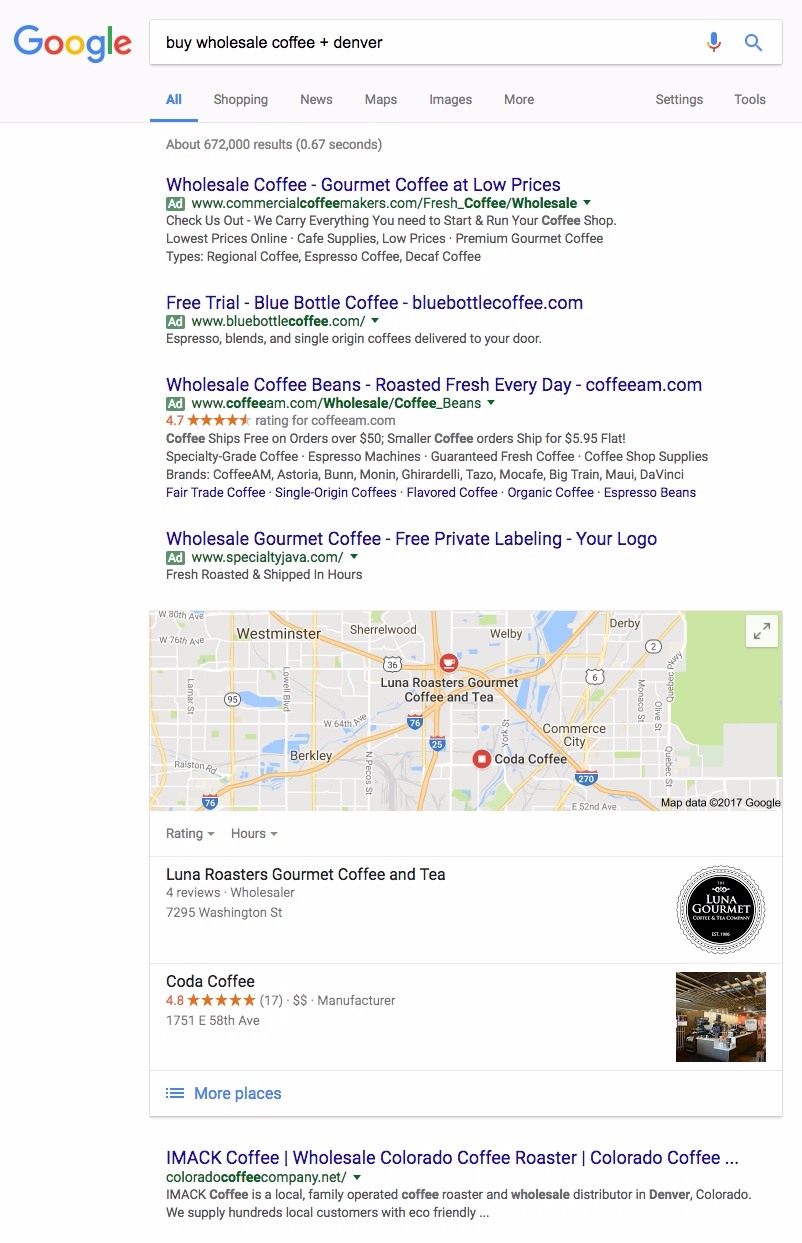This image depicts a Google search results page. In the upper left-hand corner, the Google logo is prominently displayed. Directly below the logo is the search bar, which contains the text: "Buy Wholesale Coffee Plus Denver." At the end of the search bar, a microphone icon and a magnifying glass icon are visible, indicating voice search and search functions, respectively.

Beneath the search bar lies a navigational menu, containing the following options: All, Shopping, News, Maps, Images, More, Settings, and Tools. Just below the menu, a line of text states, "About 672,000 results (0.67 seconds)," highlighting the number of search results and the quick retrieval time.

The page displays four advertised results at the top, each marked with a small green square featuring the abbreviation "Ad." The headers of these advertisements are presented in blue and read as follows:
1. "Wholesale Coffee, Gourmet Coffee at Low Prices," offering a free trial and pointing to the website BlueBottleCoffee.com.
2. "Blue Bottle Coffee, BlueBottleCoffee.com."
3. "Wholesale Coffee Beans, Roasted Fresh Everyday," linked to Coffeem.com.
4. "Wholesale Gourmet Coffee, Free Private Labeling," which invites customization with your logo.

Following the advertised results section, there is a map featuring two locations relevant to the search query. Below this map, the first regular (non-advertised) search result can be found. The overall layout and detailed elements give a clear insight into the search query and the resulting page composition.